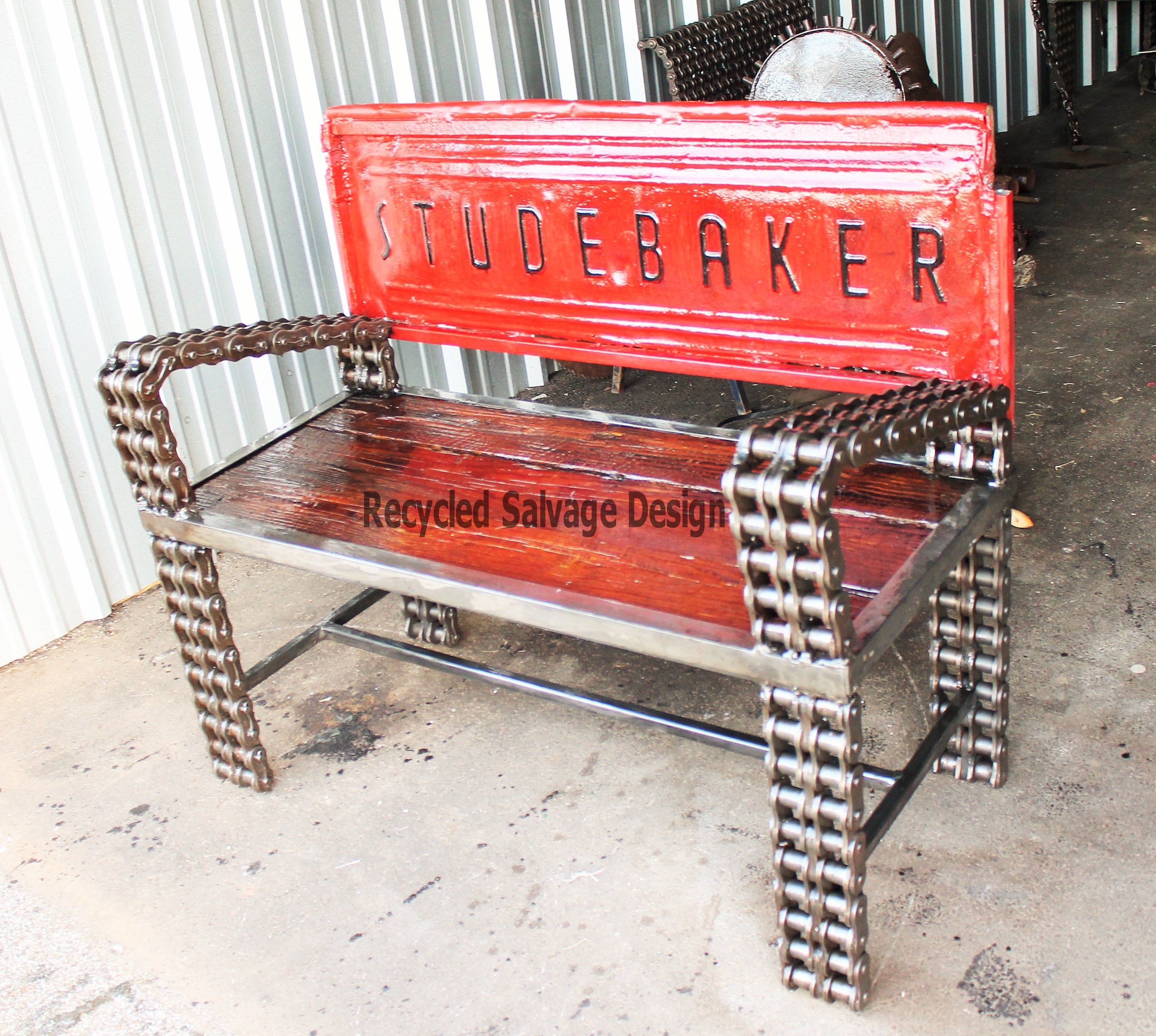The image depicts a meticulously crafted bench, designed from recycled and salvaged materials. The backrest of the bench is a repurposed part from a vintage Studebaker car, prominently featuring the "Studebaker" name in a shiny, retro red font. The seat of the bench is made of cherry-colored wood planks, surrounded by a metal rim. The armrests and legs of the bench are uniquely fashioned out of large bicycle chain links, adding an industrial aesthetic to the piece. The setting appears to be indoors, on a concrete floor, with corrugated white metal paneling in the background. Additionally, the backdrop reveals more salvage items, including a possible sunburst mirror and additional bicycle chain pieces. The photo is taken from a standing position, angled slightly downward and to the left, capturing the intriguing and innovative design of the bench.